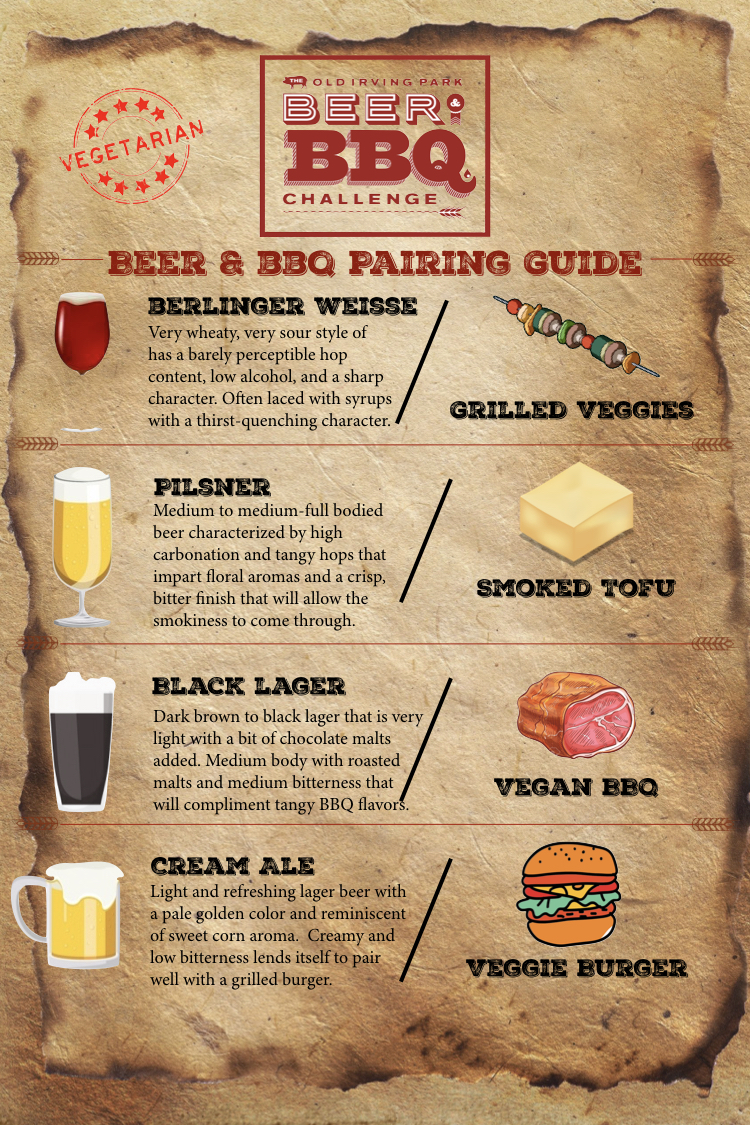The poster features a rustic, burnt-edge design on brown paper to evoke a vintage feel. At the top, a prominent red square contains the title "Beer Barbecue Challenge" in bold red letters. Above this, in smaller red text, are the words "Old Irving Park, Old Irving Park Beer Barbecue Challenge."

On the left side of the poster, a red-inked stamp marked "Vegetarian" is encircled by red stars. Below, the header "Beer and Barbecue Pairing Guide" is displayed in red letters.

The poster is segmented into four beer and food pairings, each with detailed descriptions and accompanying images:

1. **Berliner Weisse**:
   - Shows a glass of the pale, weedy, and sour-style beer with minimal hop content, low alcohol, and sharp character often sweetened with syrups. 
   - Pairs with a skewer of grilled vegetables.

2. **Pilsner**:
   - Depicts a glass of medium to full-bodied beer with high carbonation and tangy hops, delivering floral aromas and a crisp, bitter finish that enhances smokiness.
   - Pairs with smoked tofu.

3. **Black Lager**:
   - Features a glass of dark brown to black lager with chocolate malts, medium body, roasted malts, and medium bitterness that complements tangy barbecue flavors.
   - Pairs with a vegan barbecue option shown as meat.

4. **Cream Ale**:
   - Shows a beer glass with a pale golden-colored beer, light and refreshing, with a creamy, low-bitter profile hinting at sweet corn, perfect for pairing with a grilled burger.
   - Pairs with a veggie burger depicted with a bun, lettuce, tomato, and a patty.

The poster cohesively illustrates the harmonious pairing of beers and vegetarian barbecue dishes, making it an enticing guide for enthusiasts of both.